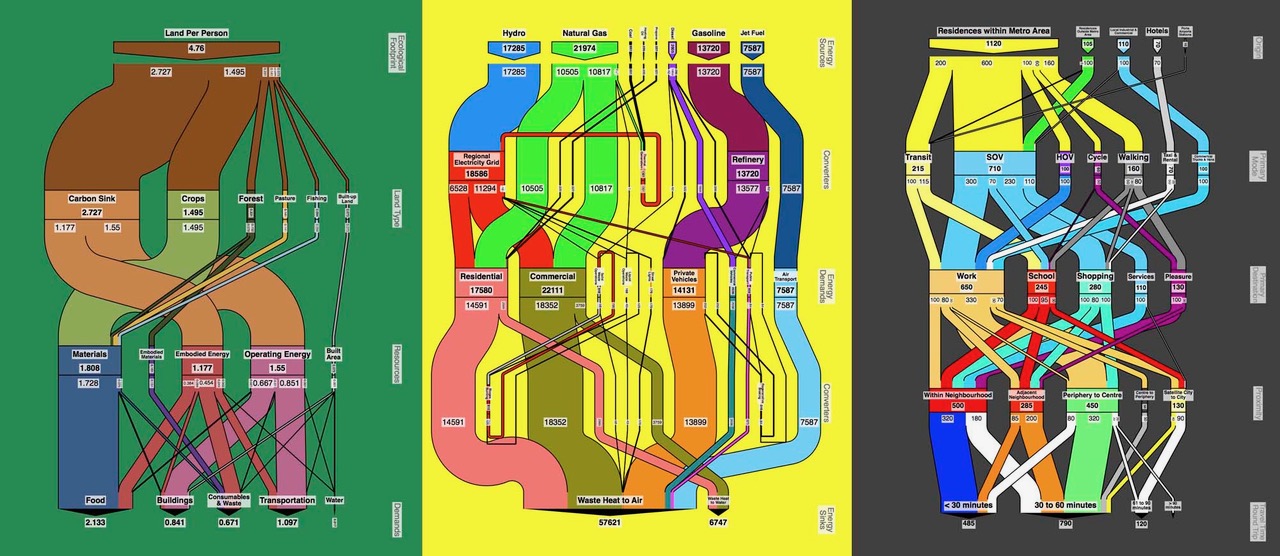The image features three side-by-side panels, each depicting an intricate network of pipes in vibrant, cartoonish colors. The first panel showcases a green background with an array of pipes in colors such as brown, red, blue, purple, and olive green. The second panel, set against a yellow backdrop, displays pipes in shades of blue, red, pink, green, brown, purple, and lighter brown. The final panel features a black background with pipes in yellow, blue, red, and green. Each pipe configuration appears to represent different systems, possibly ecological, with a detailed interplay of colors highlighting their connections and differences. The overall visual impression is one of complexity and interconnectedness within each panel's colorful, yet systematic, design.